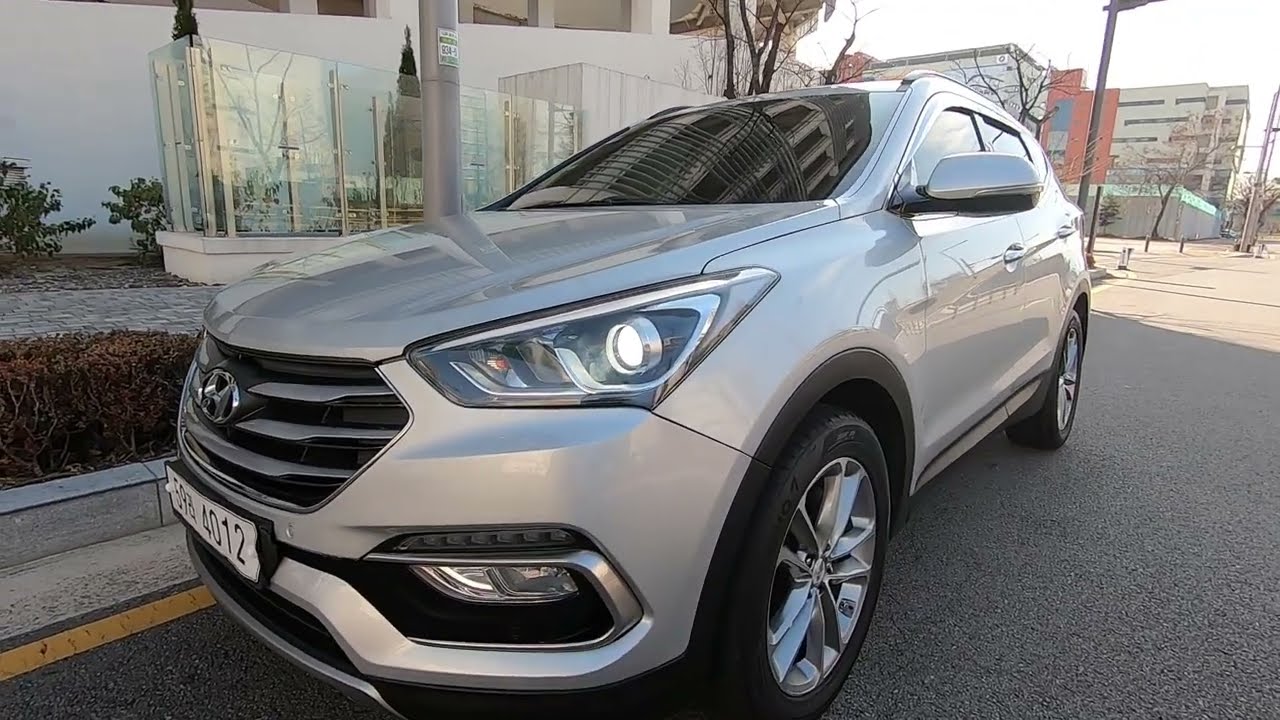The photograph captures a detailed street scene centered around a shiny, silver SUV, likely either a Honda or Hyundai, identifiable by the emblem at the front. The vehicle appears brand new, with its left front corner prominently displayed in the frame, including the left headlight and fog light, as well as the front and back wheels on the driver's side. The SUV, noticeably clean and metallic, is parked diagonally on a paved street near a yellow curb line. The license plate is partially visible, ending in the numbers 4012, and resembles a European style with white background and black numerals. The scene is set on a sunny day, although the SUV itself is in the shade, suggesting it is winter due to the bare deciduous trees lining the sidewalk. Behind the SUV are tall commercial buildings, including a white building close to the car and a beige-brick colored apartment building in the distance. A glassed-in area, likely used for outdoor seating with some greenery and trees, is situated immediately behind the vehicle. There are no other vehicles in sight.